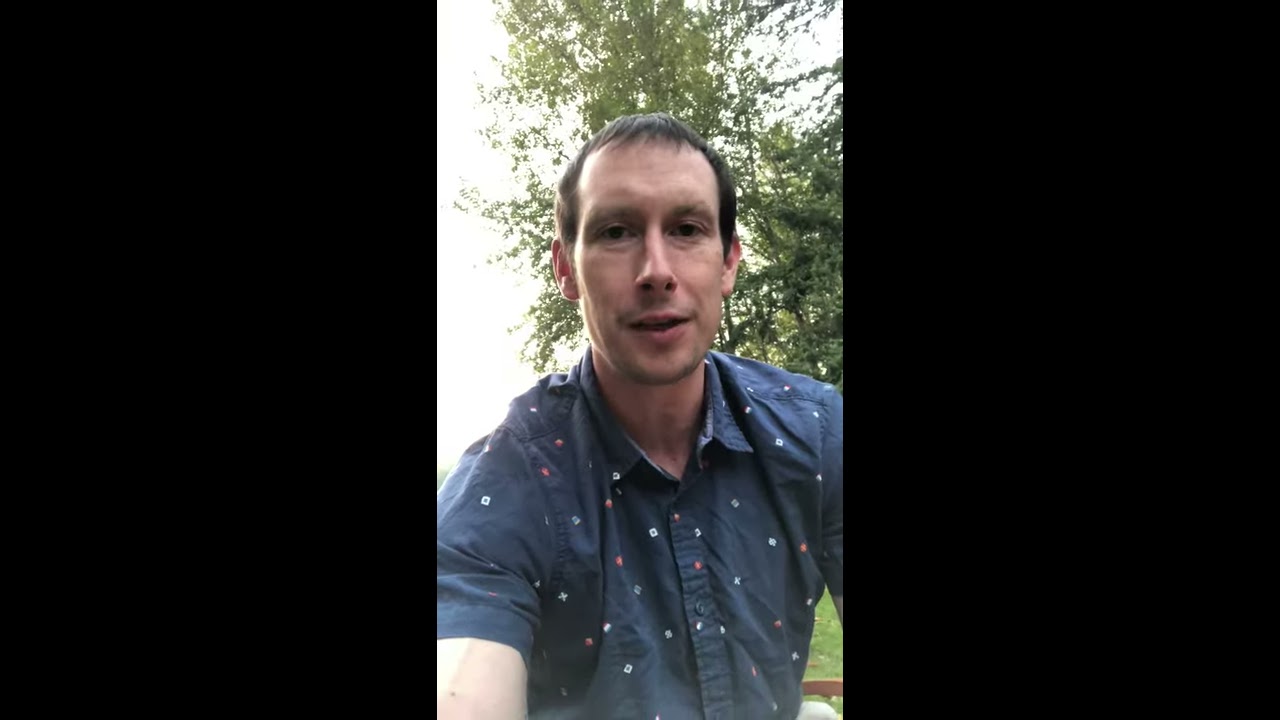A mid-to-late 30s white male with short brown, slightly receding hair is taking a selfie. He has a partially open mouth, revealing a hint of a goofy grin, and a day's worth of dark stubble. He is wearing a short-sleeve, navy blue collared button-down shirt adorned with colorful patterns that resemble squares and dots in various hues like green, red, pink, and blue. His right arm is extended, likely holding the camera. He appears thin and somewhat reserved. Behind him, abundant tall trees with bright green leaves rise against a sunny, bright sky. The sunlight streams through the branches, highlighting a grassy field in the background. He is seated on what looks like a wooden chair, and the overall scene suggests a serene, outdoor environment.